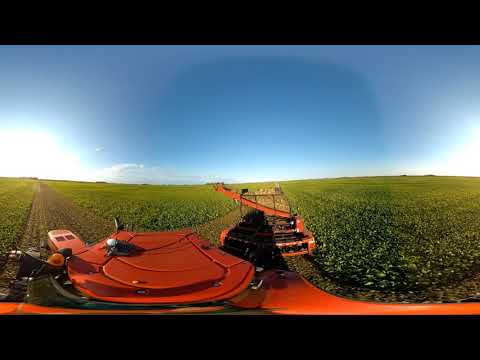This panoramic image captures a scenic, midday view of a farm field, primarily dominated by lush greenery. The image prominently features an orange harvest machine, likely a harvester or tractor, positioned towards the bottom center of the frame, just above a thick black border. The tractor is equipped with a crane-like fixture and a plowing implement that extends behind it, moving along a dirt road flanked by low-growing crops, possibly vegetables like peanuts. The expansive field stretches towards the horizon on both sides, with hints of far-off buildings dotting the distant skyline. The sky above is a perfect blue with scattered white clouds, adding to the overall serene ambiance of the outdoor setting.